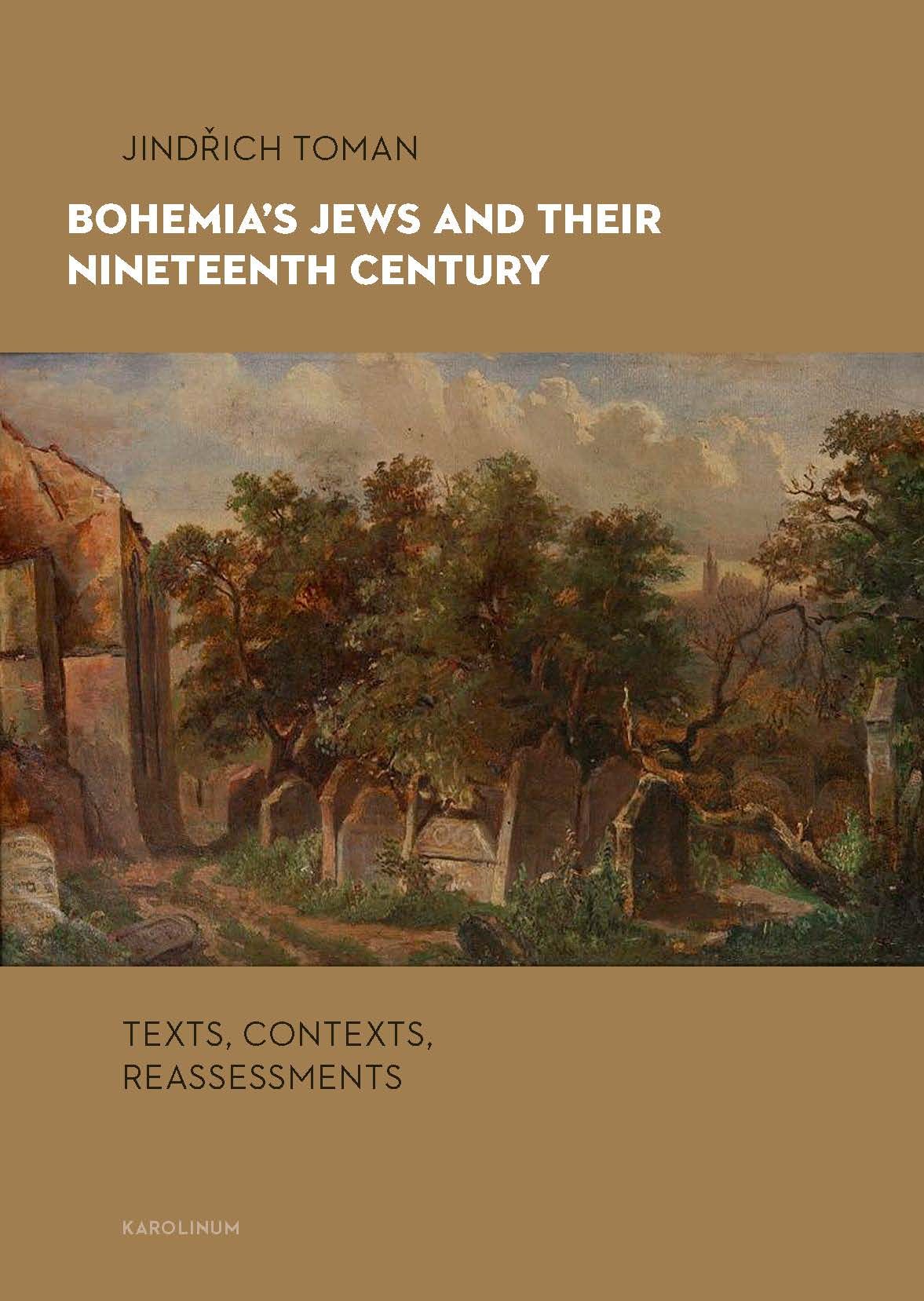The image is the cover of a book in a portrait orientation, featuring a strikingly detailed layout. At both the top and bottom thirds, the background is a brown-bronze shade. In the top section, a thin black text near the left reads the author's name, "Jindřich Toman." Below this, in bold white text closer to the left edge, is the book's title, "Bohemia's Jews and Their 19th Century," split into two lines: "Bohemia's Jews and Their" on the first line and "19th Century" on the second.

The central part of the cover showcases a watercolor painting of an ancient cemetery. This painting is rich in details, featuring various shapes and sizes of headstones surrounding trees. Some headstones have pointed tops, while others are rounded, many with faded inscriptions hinting at their age and history. The tombstones exhibit a grimy texture in shades of gray and brown. The scene is set against a backdrop of tall stones or potentially a mausoleum stretching toward a sky filled with white and gray clouds, interspersed with hints of blue. The foreground of the painting includes patches of green grass and brown dirt pathways, with some headstones toppled over. Additionally, large tree trunks and limbs stretch across the ground, and there is even a possible steeple faintly visible in the background.

In the bottom bronze section, aligned with the author's name, black text reads "Texts, Contexts," followed by "Reassessments" on the second line, both in bold. At the very bottom, in small white text and all caps, is the publisher's name, "Karolinum." This overall composition, with its detailed artwork and thoughtful text placement, suggests an academic work, potentially appealing to readers interested in historical studies or Jewish history in Bohemia.